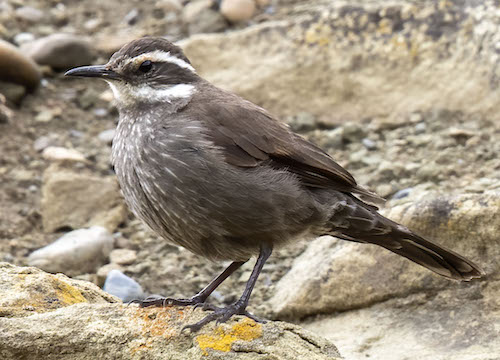The detailed, close-up photograph captures a small bird, likely resembling a sparrow, standing on a rock in a rocky coastal terrain. The bird features a mix of gray and white feathers, with distinctive white markings forming a 'C' shape on the sides of its head and eye lines. Its puffy chest exhibits white feather striations, while its slender legs support its stance. The bird's long, dark tail feathers accentuate its profile as it faces left. Its beak is narrow, thin, and dark, contributing to its sharp, attractive appearance. The bird's serene posture on the rocks emphasizes its natural habitat amidst a rock-covered gully, highlighting its subtle beauty against the rugged coastal backdrop.